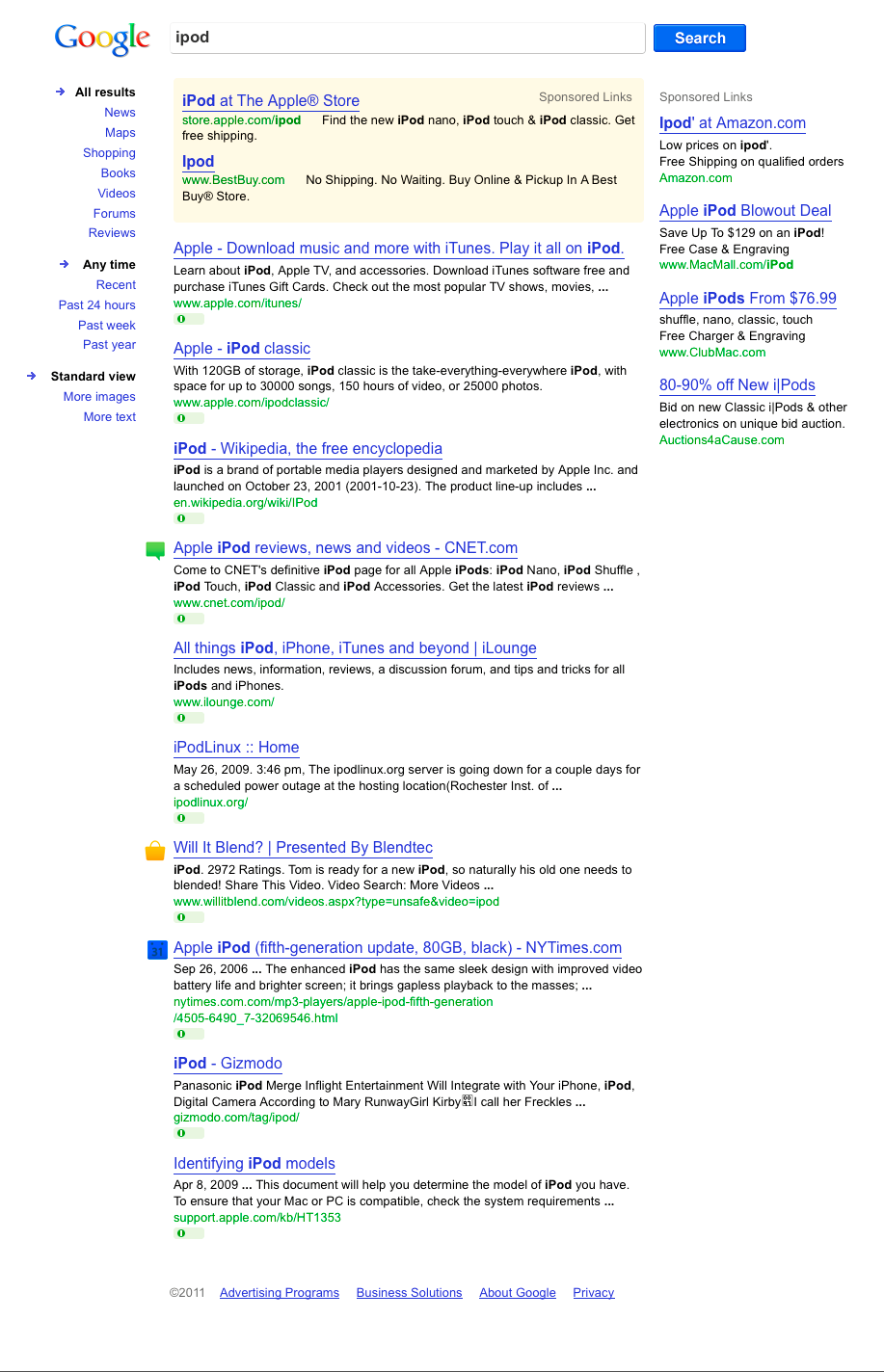The image depicts a Google search page on a mobile device, characterized by a streamlined and compressed format. The background is predominantly white.

At the top center, the quintessential Google logo appears in its vibrant colors. To the right is the elongated white search bar, containing the search query "iPod" in bold black text. Adjacent to the search bar is a blue "Search" button with white text.

Below the Google logo, a navigation bar in black font displays the option "All results," followed by a row of clickable links in blue: "News," "Maps," "Shopping," "Books," "Videos," "Forums," and "Reviews."

Under the navigation bar, a section categorizes results by time, displaying in bold black font the option "Anytime." Following this are additional time filters in blue: "Recent," "Past 24 hours," "Past week," "Past year." Another bold black option, "Standard view," is listed, followed by "More images" and "More text" in blue.

Directly below the search bar, multiple clickable links appear:
1. "iPod at the Apple store" with accompanying information.
2. Several instances of "iPod" and "Apple" links, each providing additional details when clicked.

A green square icon and a "Will it blend?" link with a yellow shopping cart icon are also present, suggesting related content. Additionally, an Apple iPod link is illustrated with a small blue calendar icon displaying the number "31."

Further down, two more clickable "iPod" links are visible. The section under "Sponsored Links" comprises four entries. 

At the bottom of the page, in gray text, is the year "2011." To the right, a series of blue, underlined links read: "Advertising Programs," "Business Solutions," "About Google," and "Privacy," concluding the search layout.

This comprehensive description captures all the elements depicted on the mobile Google search results page for "iPod," reflecting the detailed structure and various hyperlinks and icons present.